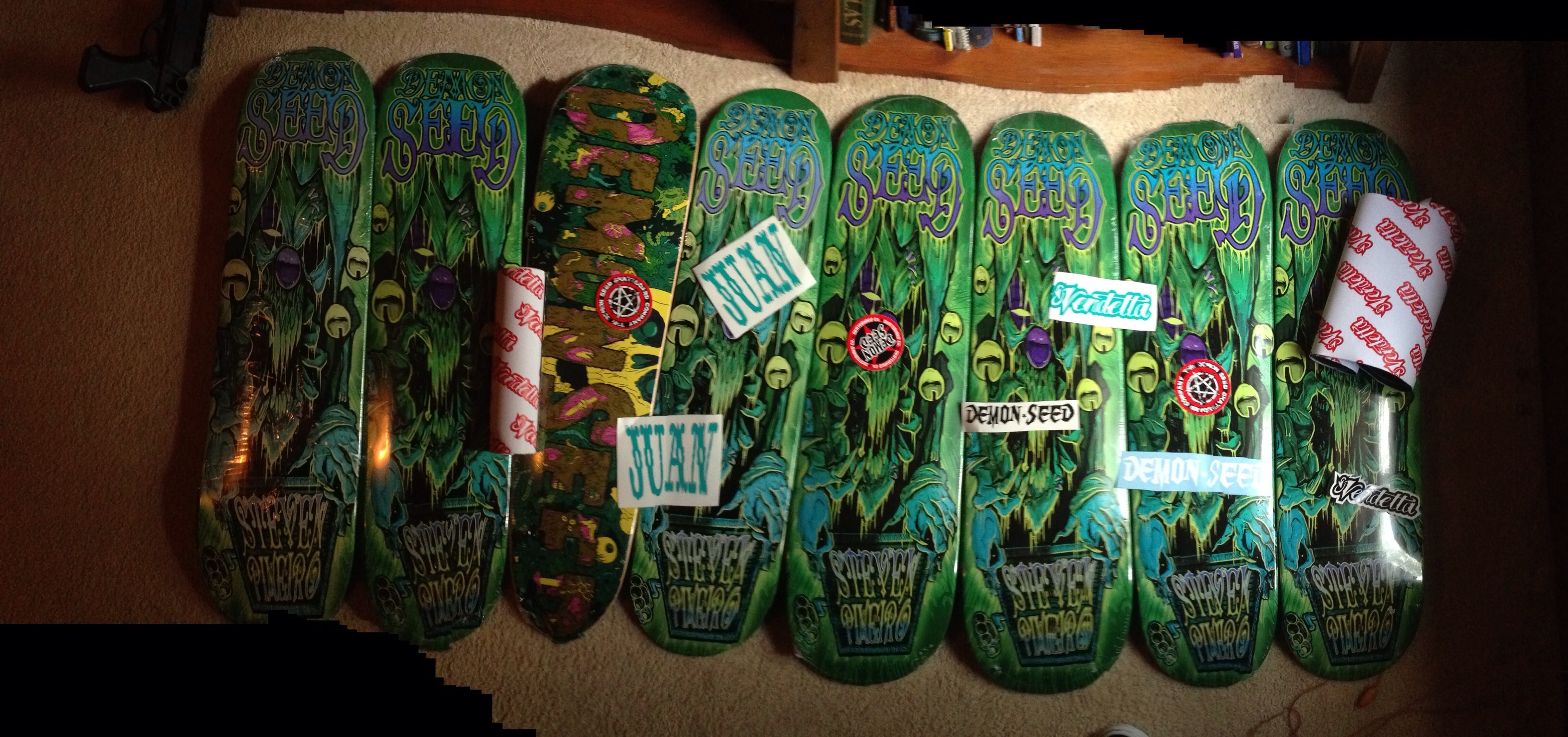The somewhat dark and poorly lit photograph depicts a row of nine rectangular-shaped stones standing on end, each resembling a skateboard deck with rounded edges. Eight of these stones have a green background, with dark, ominous stems resembling dripping black blood supporting bulb-like flowers painted in various colors, including purple and yellow. Among these, one stone distinctively features a camouflage pattern with unreadable black capital letters running vertically. The stones are arranged on a cream-colored fabric, bordered by a darker brown wooden surface. In the center of the row, one stone stands out with a floral design that says “D.E.M.” in pink lettering from top to bottom. Adjacent to these stones are numerous identical stones painted with blue along the top edge and a gray stone-like pattern on the bottom, bearing white labels with blue "San Juan" inscriptions. A piece of white paper with diagonal red writing hangs off the far right edge of the scene, adding to the clutter of souvenirs.